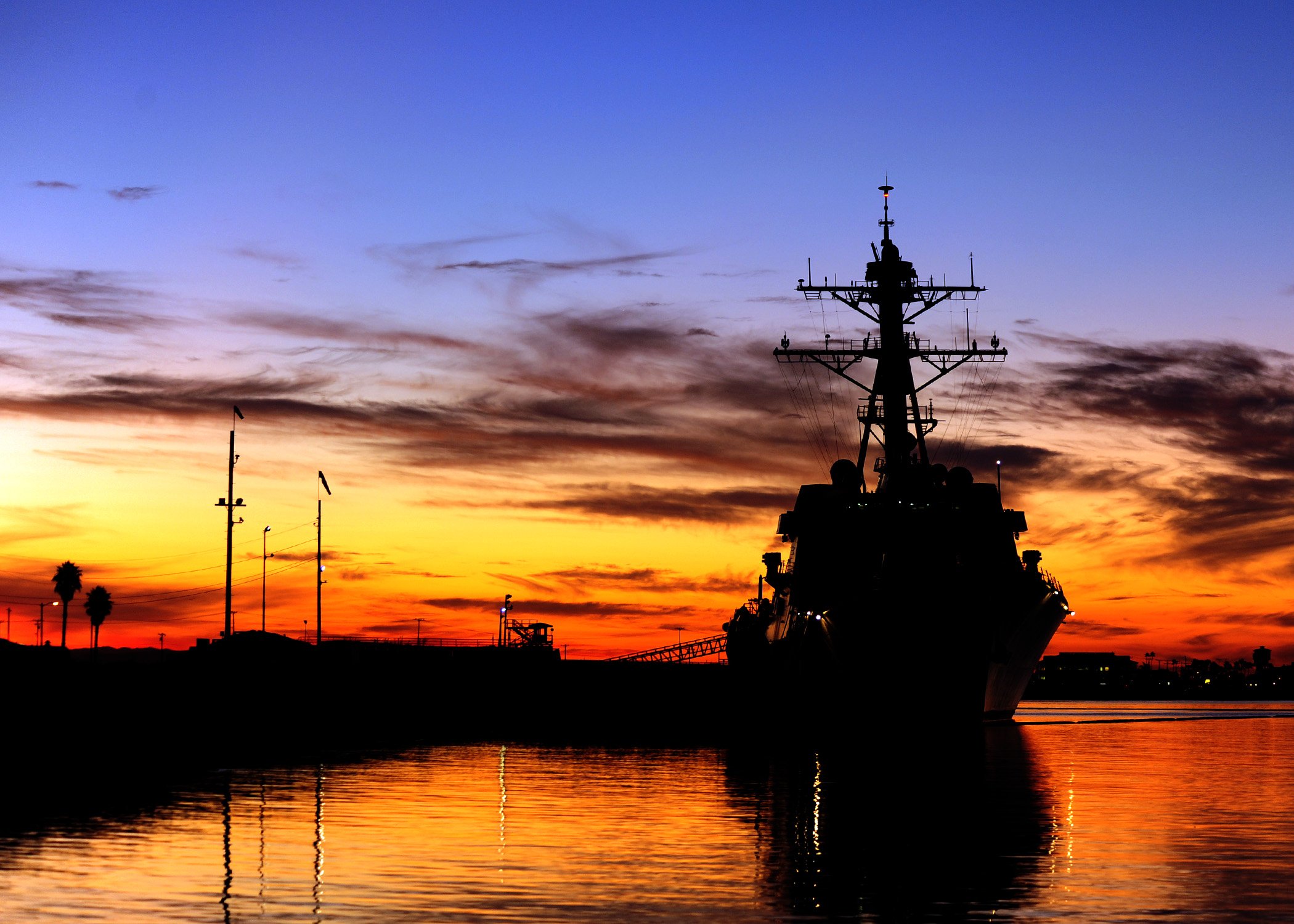In this captivating sunset photograph, taken by the waterfront, the scene is dominated by the silhouette of a large navy battleship anchored at a port. The vessel, featuring tall masts with dual extenders and multiple levels equipped with satellite and radio antennas, stands prominently against the vivid sky, casting a significant shadow on the calm waters below. The water mirrors the sunset's warm hues, transitioning from a deep red at the horizon to a bright yellow-orange, and finally to a serene blue at the sky's highest point. Wispy clouds punctuate the sky, growing darker as they descend. On the left, electrical poles and a palm tree-like silhouette add depth to the composition. In the distance, faint lights hint at a distant hilly area with possible houses or businesses, completing this serene yet striking maritime scene.